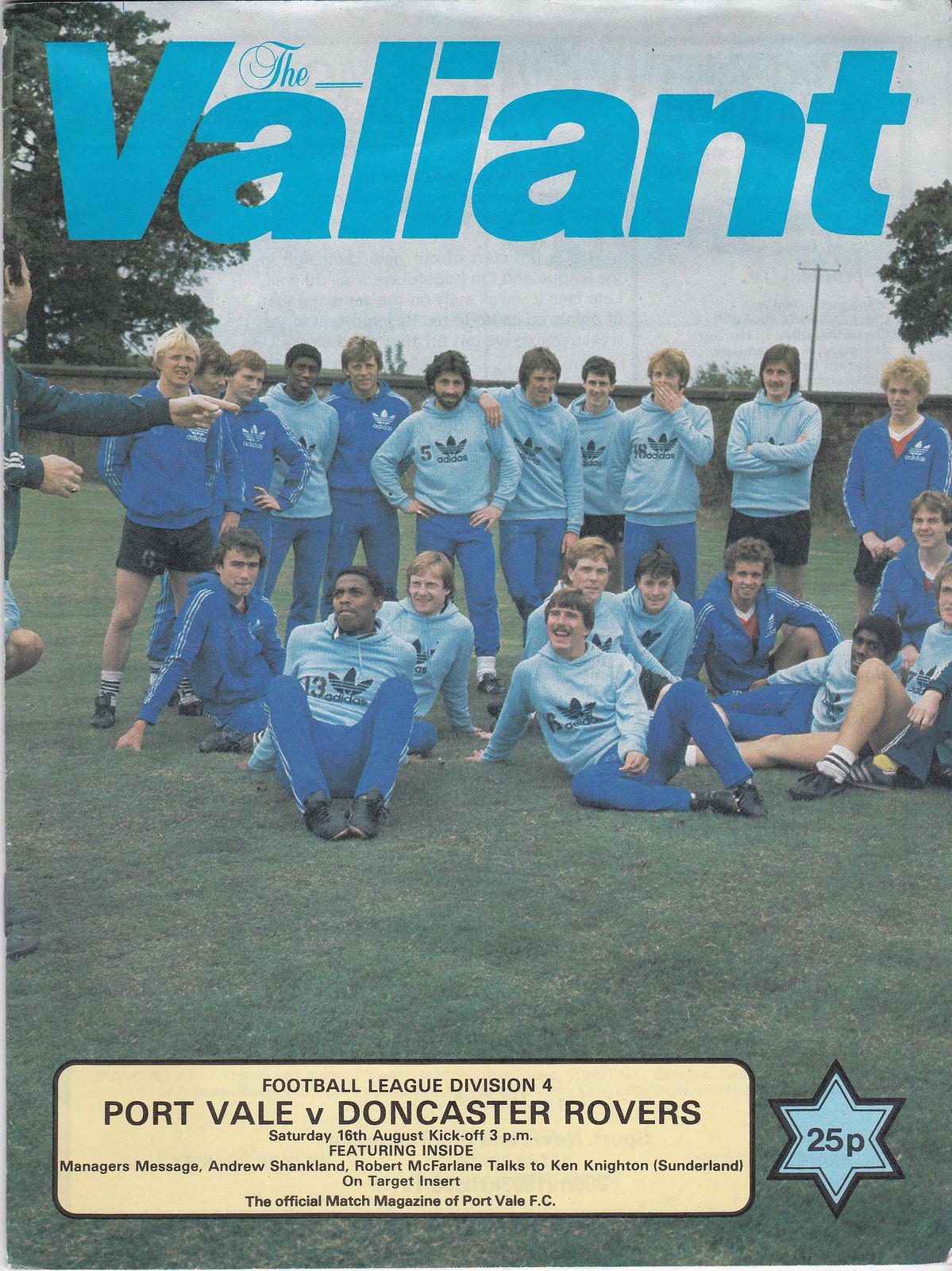The cover image for a soccer program prominently features the title "The Valiant" in large, bold blue letters at the top, with the word "The" in smaller text above the first "A" in "Valiant." Beneath the title is a team photo depicting two rows of players in blue and light blue warm-up gear. The players' attire includes long sleeve sweatshirts—some lighter blue with a black Adidas logo at the center and some darker blue zip-up hoodies with a white Adidas logo on the breast pocket. The photo features a row of men standing in the back while a row of young men are seated or crouched on the grass in front, all smiling, some playfully goofing off. On the left side of the image, a figure, likely the coach, dressed in a dark blue jacket, is seen pointing to the left with his left hand. At the bottom of the image is a yellow text box with the details: "Football League Division IV, Port Vale vs. Doncaster Rovers, Saturday, August 16th, kickoff at 3 p.m." Additional text mentions segments such as the manager's message, an interview with Andrew Shankman and Robert McFarlane talking to Ken Knighton of Sunderland, and an "On Target" insert. To the right of this text box, a six-pointed star marks the price as 25p.